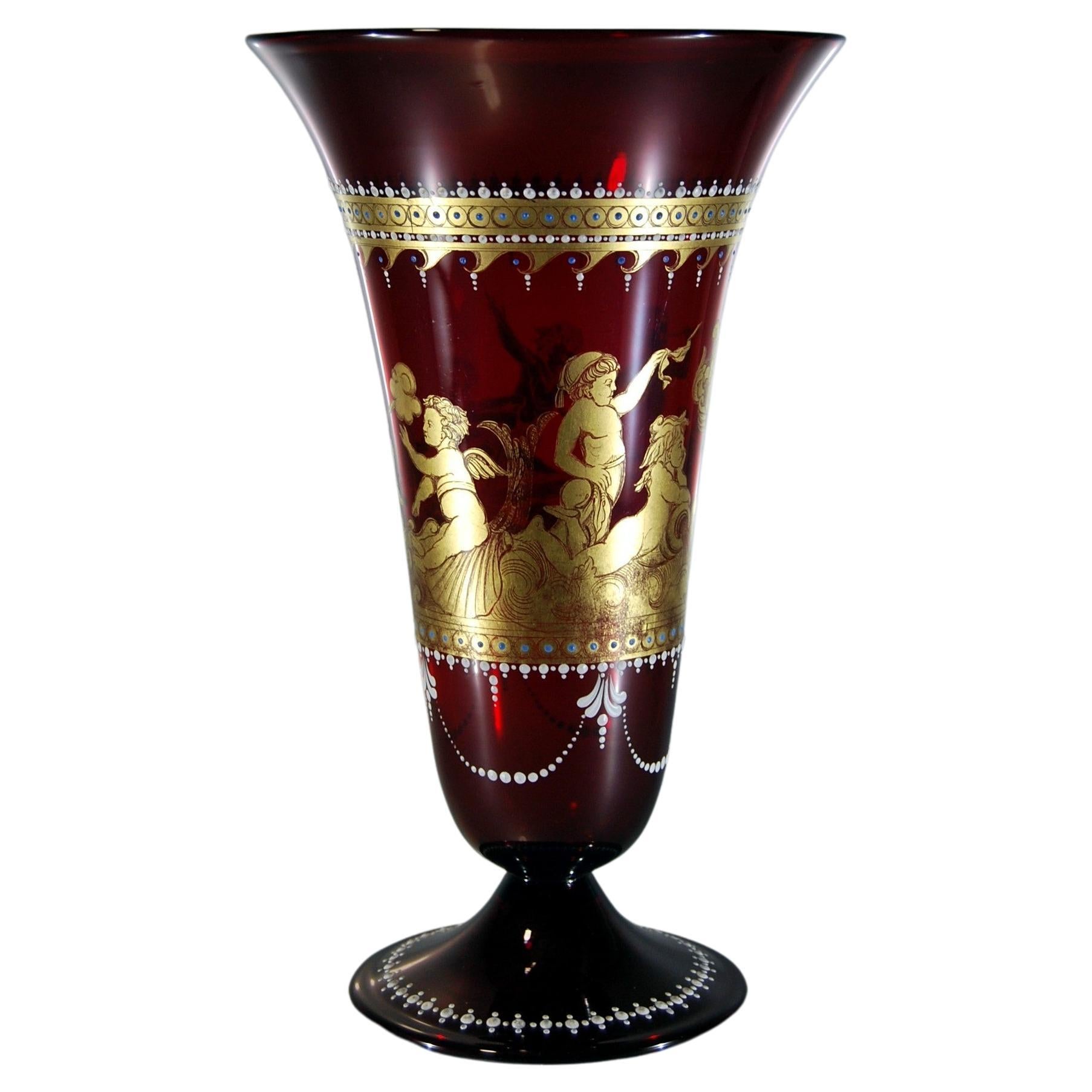The photograph features a tall, elegant vase placed against a completely white background and surface, making the detailed artwork on the vase stand out prominently. The vase, appearing to have a Grecian influence, is fashioned from dark ruby-red glass, which is somewhat translucent, allowing the intricate designs to reflect through. The vase has a round base adorned with a white diamond pattern circling it. Slightly above this base, a white garland-like design drapes in loops, adding a delicate touch before the vase narrows and then gracefully flares out into a tulip shape, culminating in a wider flange at the top.

The central portion of the vase is embellished with an elaborate golden inlay depicting cherubic figures, possibly shepherd angels or cherubs, engaged in various activities, creating a narrative element to the piece. This middle section is bordered by a golden band adorned with concentric circles. Additional white designs echo this motif, appearing both below the cherubic scene and again around the uppermost rim, providing a balanced visual harmony to the ensemble. The vase's detailed artistry and composition make it a striking and cultured piece, suitable to be displayed prominently on a shelf.